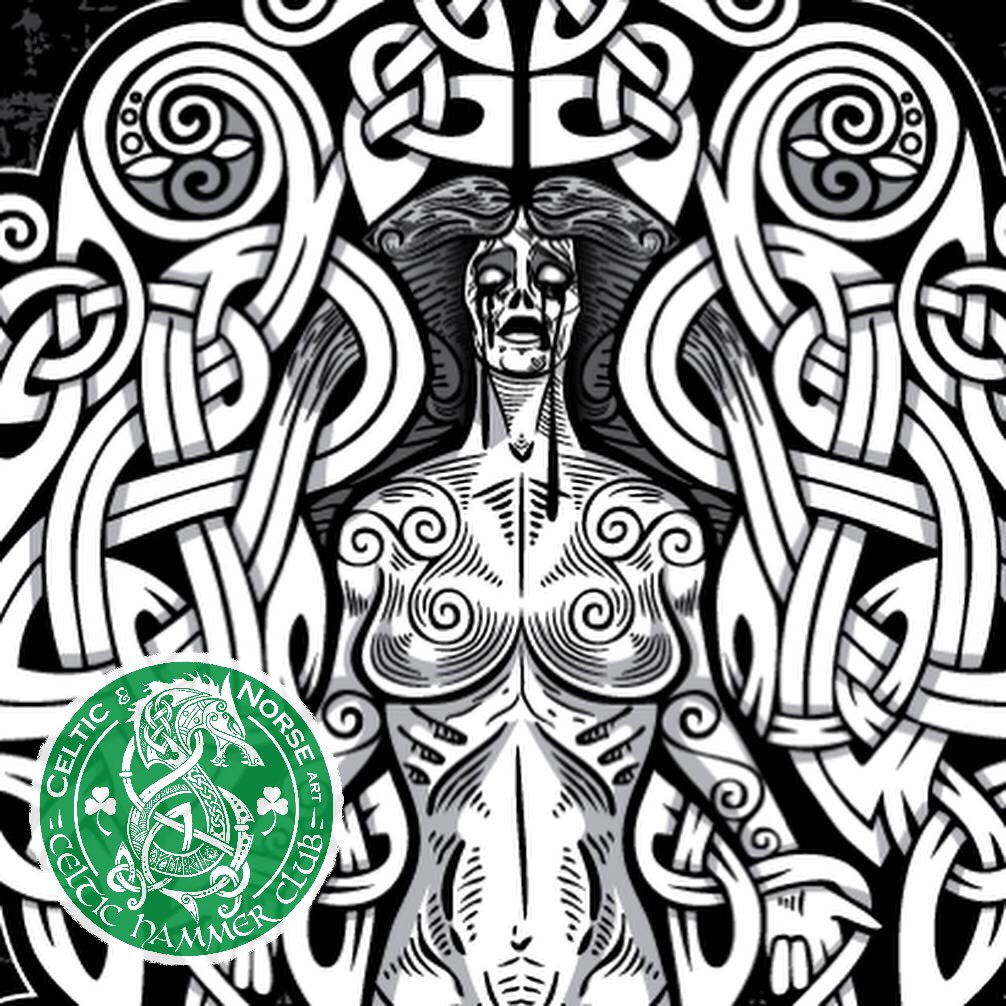The black and white image appears to be computer-generated and depicts a highly detailed and dramatic scene. At the center is an illustration of a naked woman, who is crying tears of dark blood from pupil-less white eyes. Her body is intricately adorned with Celtic tattoos. Surrounding her is a sophisticated design of ribbon-like, braided patterns that weave in and out in a circular motion, almost resembling bandages or Nordic-style braiding. In the bottom left corner of the image, there is a translucent green circular logo featuring a white dragon, and adorned with clovers on either side. This logo contains text that reads "Celtic and Norse Art, Celtic Hammer Club." The entire composition exudes a dynamic and intense atmosphere, blending elements of Celtic and Norse artistry.